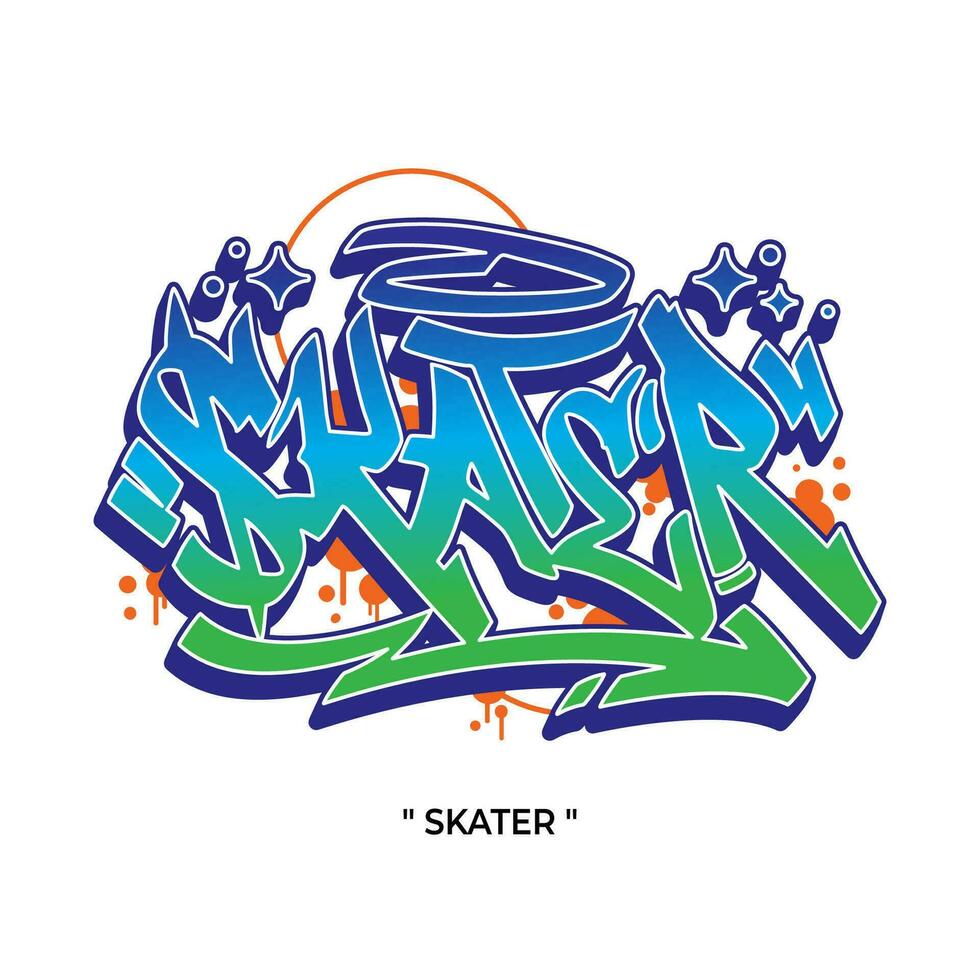The image is a vibrant and dynamic piece of graffiti art set against a white background. Central to the image is the word "skater," stylized in a unique graffiti font where the 'S' resembles a dollar sign. The text exhibits a gradient color scheme that transitions from dark blue at the top, through a lighter blue in the middle, and finishes with green at the bottom. Flanking the word "skater" are quotation marks in a similar gradient style, positioned just before the 'S' and after the 'R'. Above the word, a large, outlined orange circle reminiscent of a halo hovers over the letter 'T'. The backdrop features an assortment of orange splashes and dots, evoking the appearance of dripping paint, with some in solid circles and others partially filled. Adorning the top, stars and various circular elements in shades of purple enhance the design. Beneath the graffiti, the word "skater" is reiterated in black capital letters, encased in quotation marks.